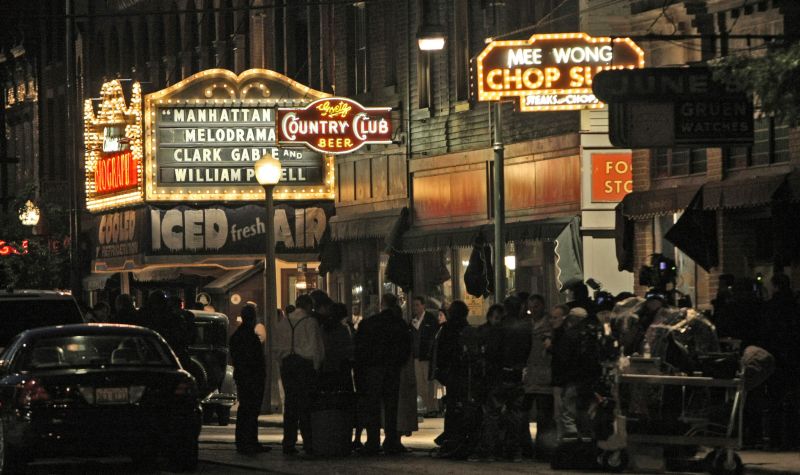This nighttime cityscape photograph captures a bustling street scene, likely in New York, focusing on an old theater with a glowing marquee that reads "Manhattan Melodrama" starring Clark Gable and William, though the last name is partially obscured. The well-dressed crowd, their silhouettes visible in the soft yellow marquee light, appears to be either waiting for the show to start or for tickets to be sold. Nearby, there are several distinctive neon signs, including "Country Club Beer" and "Mee Wong Chop Suey," adding splashes of red to the predominantly dark tones of black and gray. The framed shot also reveals a professional video camera set up, suggesting a movie scene being filmed, with vintage cars parallel parked along the street. The buildings, characterized by their brick and wood siding, invoke a classic New York ambiance, enhanced by an additional sign that reads "June Green Watches." Overall, the photograph richly details urban nightlife and culture, centered on the theater and its expectant crowd.